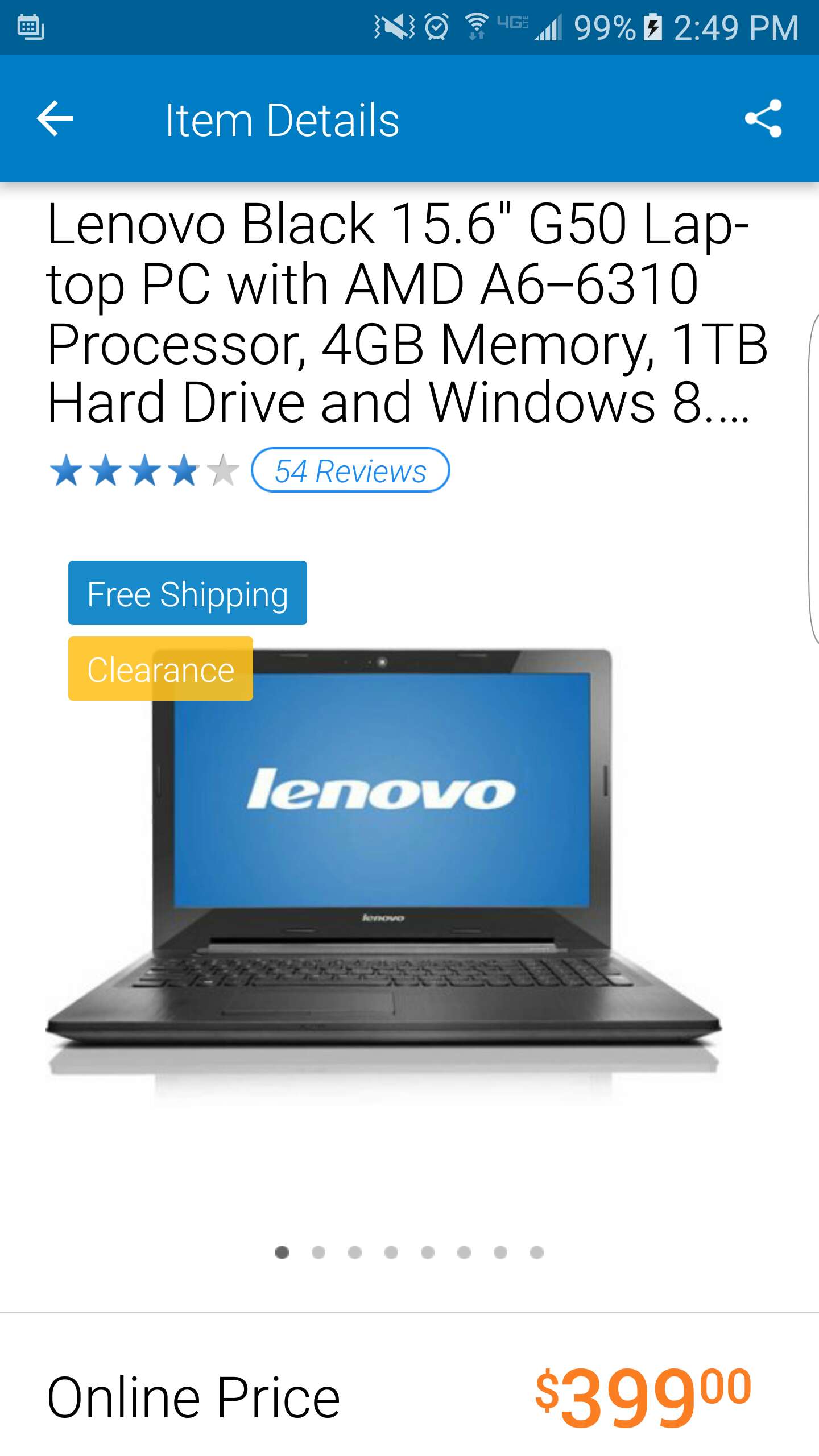A screenshot displays the item detail of a Lenovo laptop. The laptop itself is black, featuring a blue screen prominently showing the following information: "Lenovo," "Free Shipping," "Clearance," "Online Price: $399.00." The laptop also boasts a customer rating of 4 out of 5 stars, based on 54 reviews.